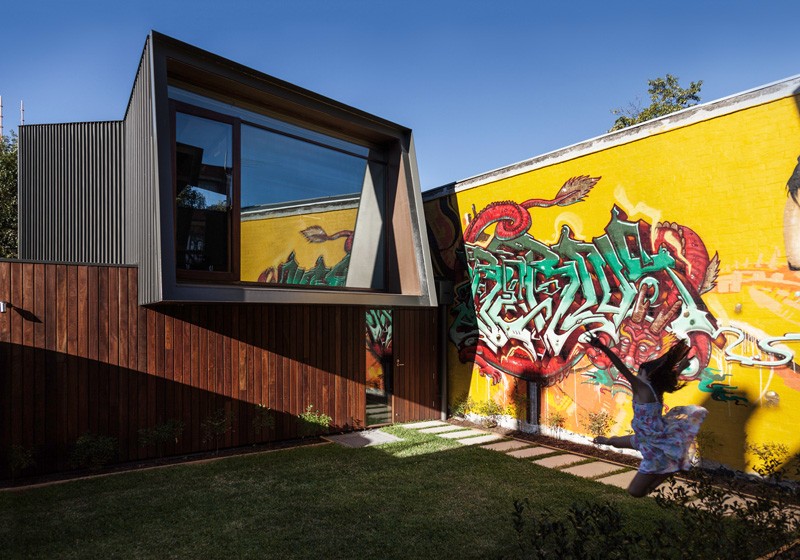This vibrant image captures a sunny day under a blue sky, showcasing a modern home with a large reflective window on the second floor. In the foreground, a lively scene unfolds with a young girl, wearing a pink dress and sporting brown hair, energetically jumping up and down on a green lawn. Behind her, a striking yellow wall serves as the canvas for an intricate and colorful piece of graffiti art featuring a red demon with yellow eyebrows and brown horns, accented with green graffiti elements.

The yard also includes a wooden mahogany fence leading to the base of the home, where a door can be accessed via several stone steps embedded in the grass. Sunlight bathes part of the scene, enhancing the lively and engaging atmosphere of this unique, modern setting.